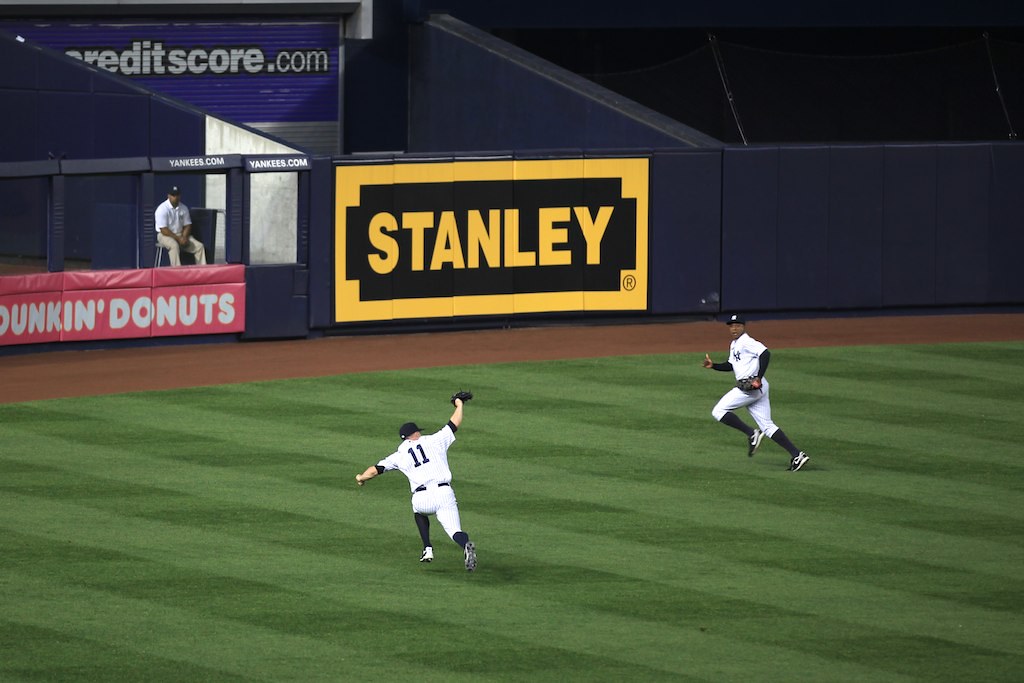This photograph captures a dynamic scene at Yankee Stadium with two baseball players in full motion on a meticulously mowed green field, the lines of which are visibly precise. Both athletes are wearing the iconic white New York Yankees uniforms with long navy blue sleeves, socks, and matching dark caps. The player to the left, identified by the number 11 on his back, is mid-stride alongside his teammate, racing towards the outfield wall. On their hands, they each have catcher's mitts, ready for action. The stadium's outfield wall prominently features a red “Dunkin’ Donuts” banner in white font, and a yellow “Stanley” banner with a bold black border and a second, finer yellow border. Additionally, a smaller advertisement for creditscore.com is visible on the barricades, which are colored in navy blue. The edge of the field transitions into a section of clay dirt, marking the boundary of the grassy expanse. A person can be seen seated in the background, attentively observing the unfolding play.